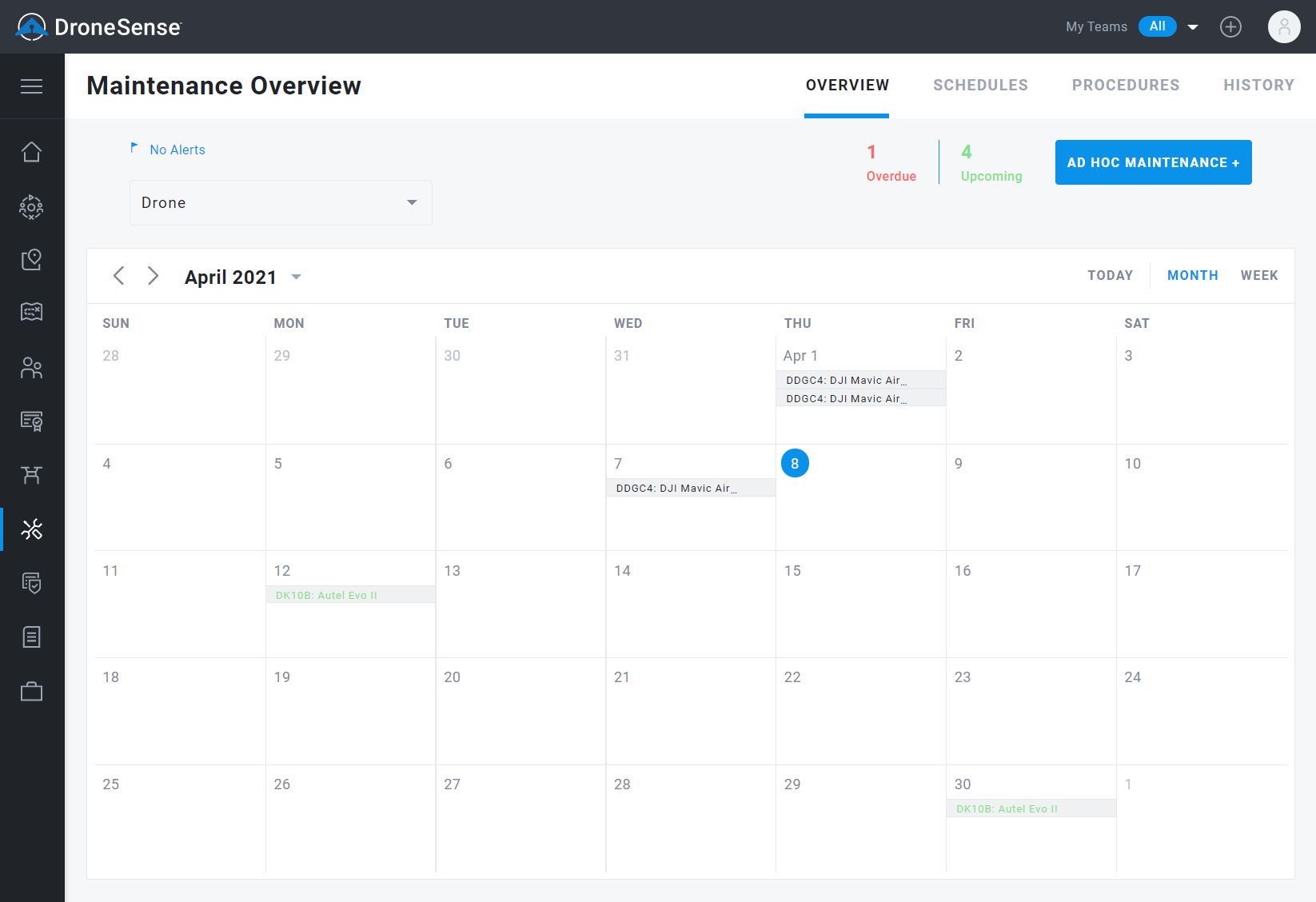This image is a screenshot from the DroneSense platform. In the upper left-hand corner, the DroneSense logo appears in white font, accompanied by a symbol resembling an 'A' enclosed in a circle. A vertical menu bar featuring various icons is situated along the left-hand side of the window. The icon selected is a crossed screwdriver and wrench, signifying the "Maintenance Overview" section. Dominating the central part of the screen, the main window is focused on the Maintenance Overview dashboard. Positioned at the top left-hand corner within this section, the heading "Maintenance Overview" is prominently displayed against a white background. Below the heading, a calendar for April 2021 is visible, highlighting scheduled maintenance tasks. Specifically, maintenance activity is noted for Thursday, April 1st.